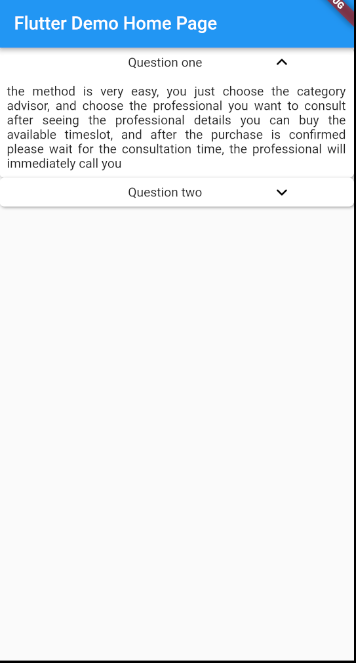A detailed caption for the image could be:

"This screenshot captures a section of the 'Flutter Demo' homepage, featuring a customer inquiry and a response. At the top left corner, 'Flutter Demo Homepage' is prominently displayed. Below, under the subheading 'Question 1,' a clear and concise method for booking a consultation is outlined: 'The method is very easy. You just choose the category, select the advisor, review the professional's details, and purchase an available time slot. After the purchase, wait for the scheduled consultation time. The professional will then call you immediately.' Beneath this detailed guide, there appears to be another section labeled 'Question 2,' possibly featuring a drop-down menu for additional inquiries."